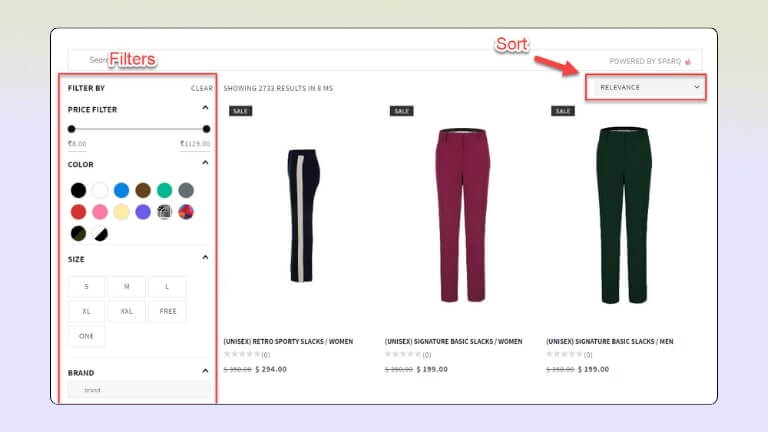The image depicts an online shopping interface for purchasing pants. The website features a detailed filter system to assist users in narrowing down their choices. At the top, there is a clear indication that filters have been applied, particularly for price, which can be adjusted via a toggle bar ranging from $0 to $1,129. Below the price filter, a color palette is displayed, featuring six circles per row across two rows, followed by a final row with two circles.

Size options are also available, including small, medium, large, extra-large, and XXL, as well as a 'Free' size. There is a section for filtering by brand, with a search field to the right. The results section shows that 2,732 items have been found, with a rendering speed of 8 ms.

To the right of the results, there is a dropdown menu under a 'Relevance' label, highlighted by a red rectangle and arrow pointing to the "Sort" option. The font style for "Sort" mirrors that of the filters section at the top, suggesting an emphasis for educational purposes. Additionally, red boxes around all the filter options further highlight their importance and usability.